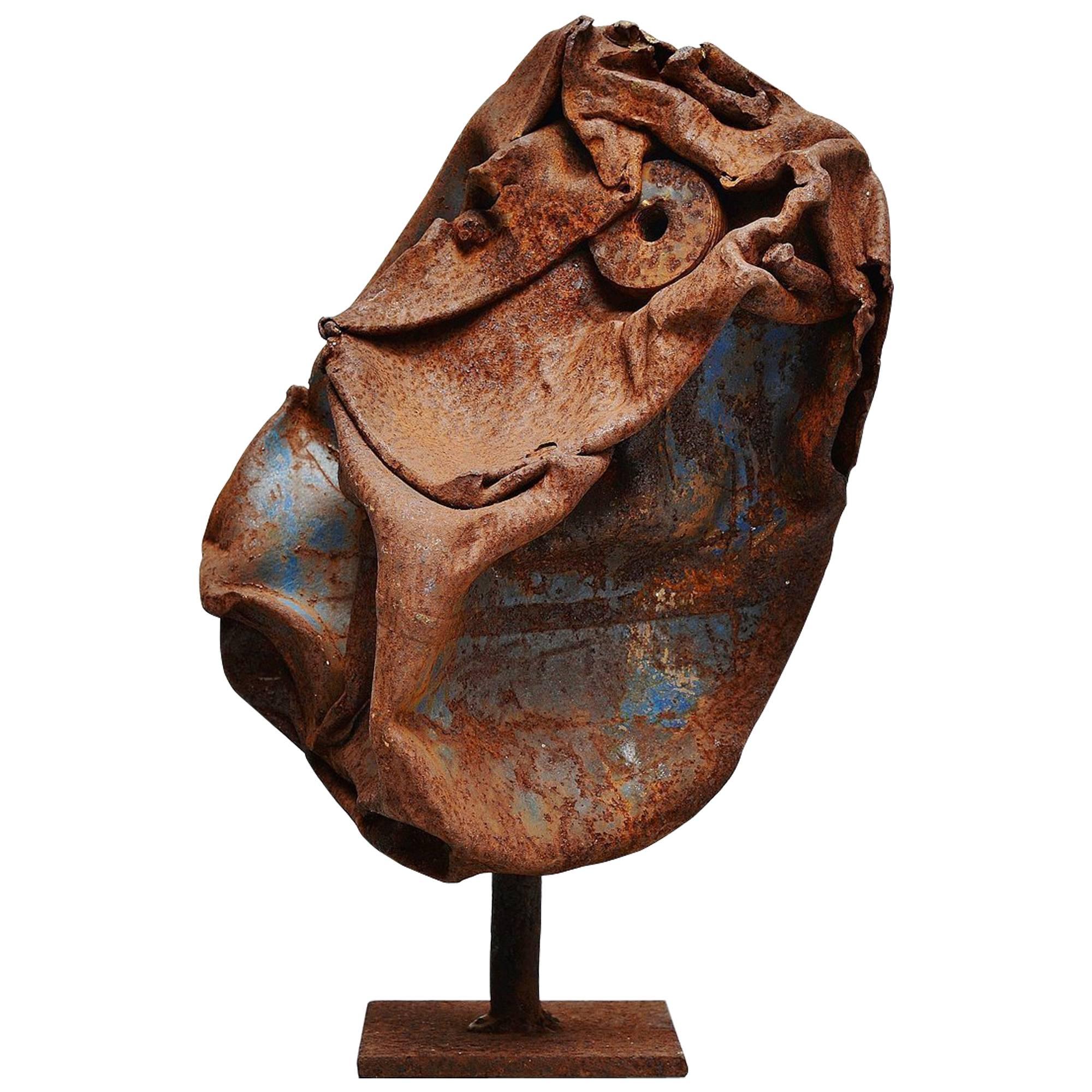This is a professionally shot, full-color photograph of a staged sculpture displayed against a plain white background. The sculpture stands on a square wooden base, dark-stained with a cylindrical rod rising from its center. Atop the rod, the focal point of the piece is a mangled, oval-shaped mass of rusty metal. The sculpture, evoking the visage of either a bird or a dinosaur, features what seems to be an eye made from rusty washers situated near the top right of the structure. Patches of the original blue paint are visible amidst the pervasive rust, specifically on the lower left, lower center, and upper right sections of the sculpture. The overall form is cluttered and crushed, creating an impression of aged, weather-beaten deterioration. The piece portrays a sense of abstract, almost primal art, leaving its precise origins and meaning open to interpretation.